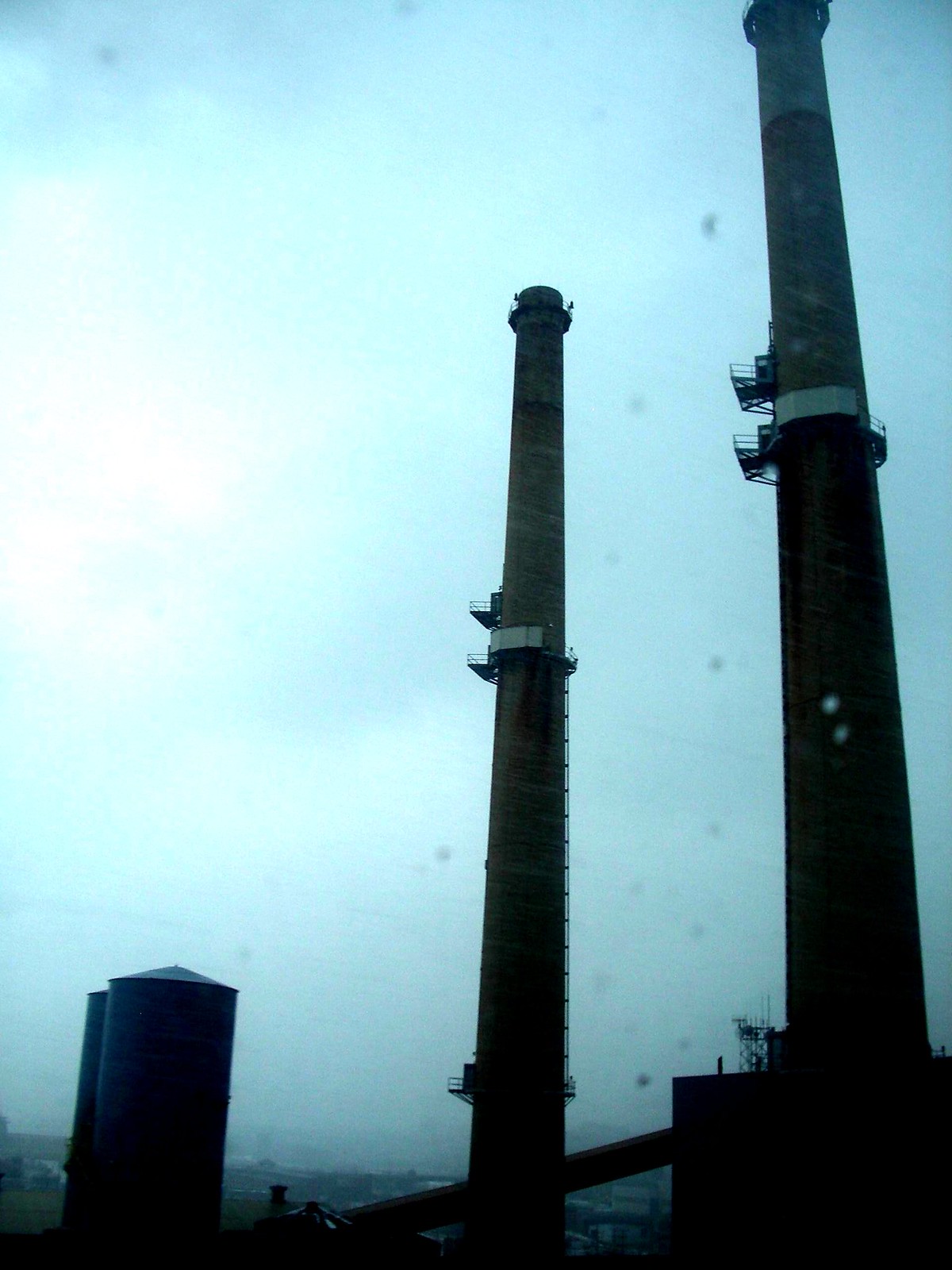The image depicts a close-up of two towering smokestacks against a hazy, blue-gray sky, evocative of the cover of Pink Floyd's "Animals" album but without the iconic flying pig. The smokestacks, made of dark brick and featuring several maintenance walkways and white stripes around their midsections, rise prominently in the composition. The sky is clear with minimal clouds, giving an impression of early morning or late evening, with sunlight filtering through a thin layer of smog. To the left, additional industrial structures are visible, including two large silos and a smaller building, reinforcing the factory setting. The entire scene combines concrete and brick elements, capturing the grit and industrial ambiance of the site.